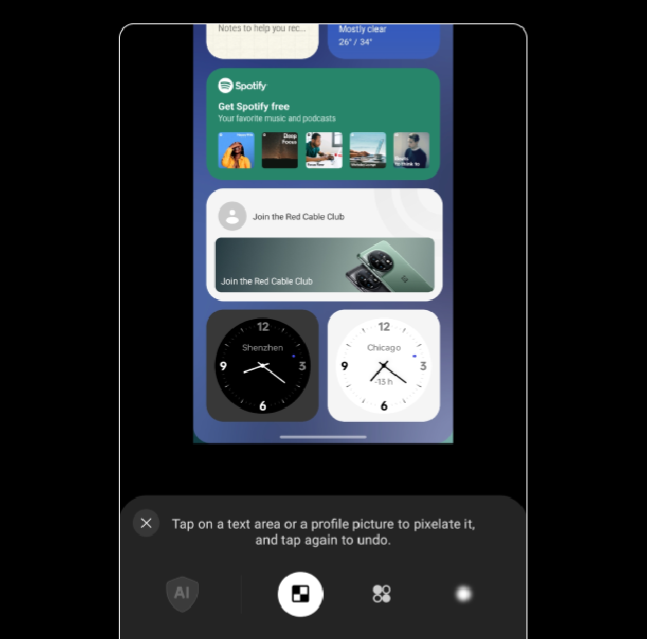Here's a detailed, cleaned-up description:

The image features a black background with a prominent square outline positioned centrally, marked on the left, right, and top edges. Within this square, there is a green button displaying the text "Get Spotify Free," with a window opening beneath it that reads "Spotify."

Below this, five thumbnails are arranged in a row. The first, third, and fifth thumbnails depict images of people, while the second and fourth thumbnails are indistinguishable in their content. Under the thumbnails, there's text that reads "Join the Red Something Club," though the exact wording might be obscured.

Further down, the image shows two clocks. The clock on the left is set inside a dark gray box, and the clock on the right is inside a white box. Both clocks display the same time, approximately 7:22.

At the very bottom, a message instructs the user to "Tap on a text area or profile picture to pixelate it and tap again to undo."